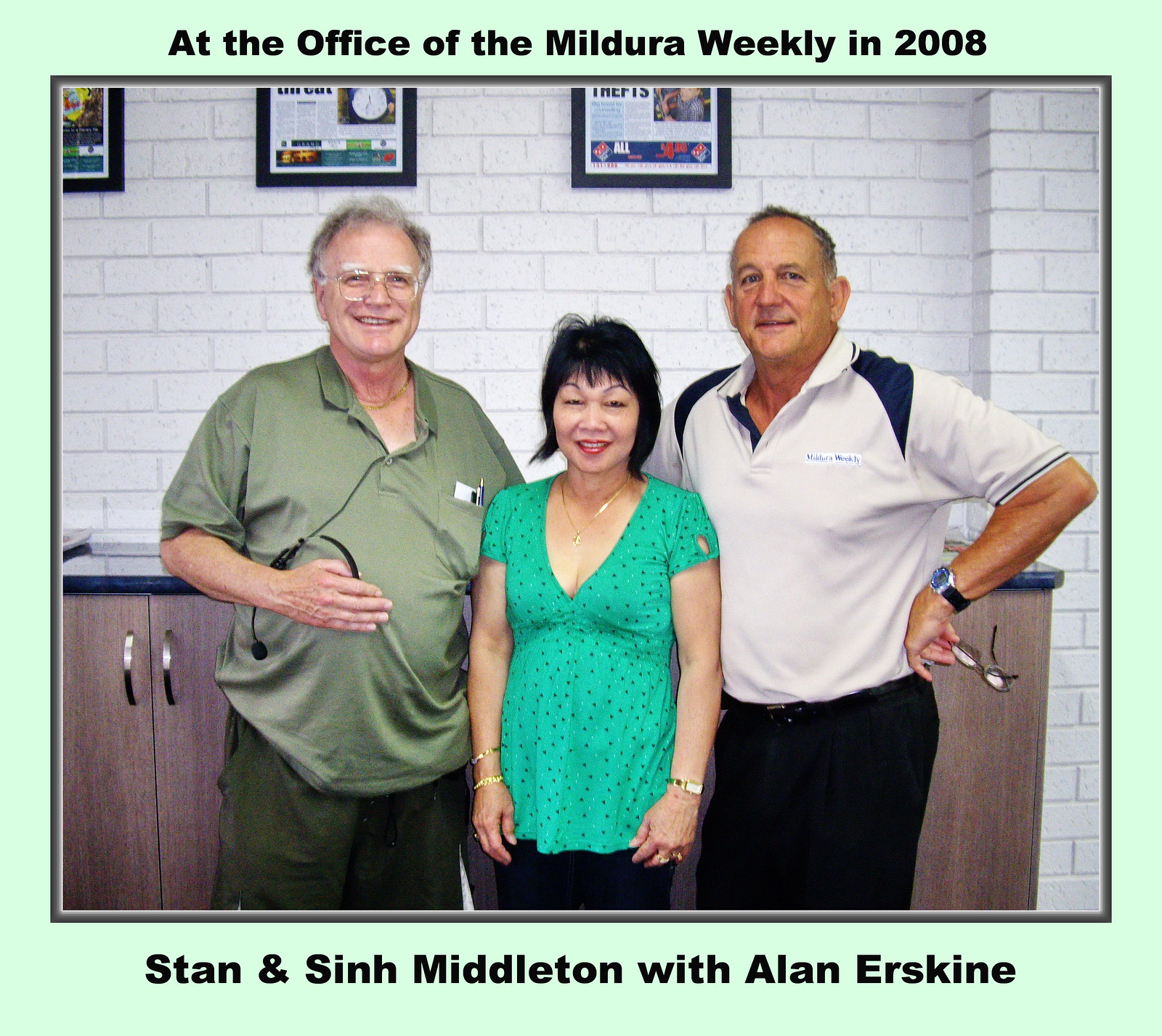This photo, taken at the office of the Mildura Weekly in 2008, features three individuals standing together in a casual, office-like setting. On the left, there's an older Caucasian man in his early 60s with thinning, gray hair. He is smiling slightly and wears glasses with very light-colored frames, making them nearly invisible unless you catch the reflection on his clear lenses. He is dressed in a loose, green short-sleeved collared shirt. Standing next to him in the middle is an Asian woman of shorter stature, appearing to be in her 50s. She is wearing a light mint green tunic-style shirt with black slacks. To her right is another Caucasian man, slightly tanner, and similarly aged in his early 60s. He has his outer arm on his hip and is holding eyeglasses. He is dressed in a white button-up polo shirt with blue accents on the shoulders and is also wearing black slacks. Behind them, there is a desk, cupboards, and a white brick wall with signs on it, contributing to the professional yet relaxed atmosphere of the office, enhanced by the smiles and casual outfits of the subjects.